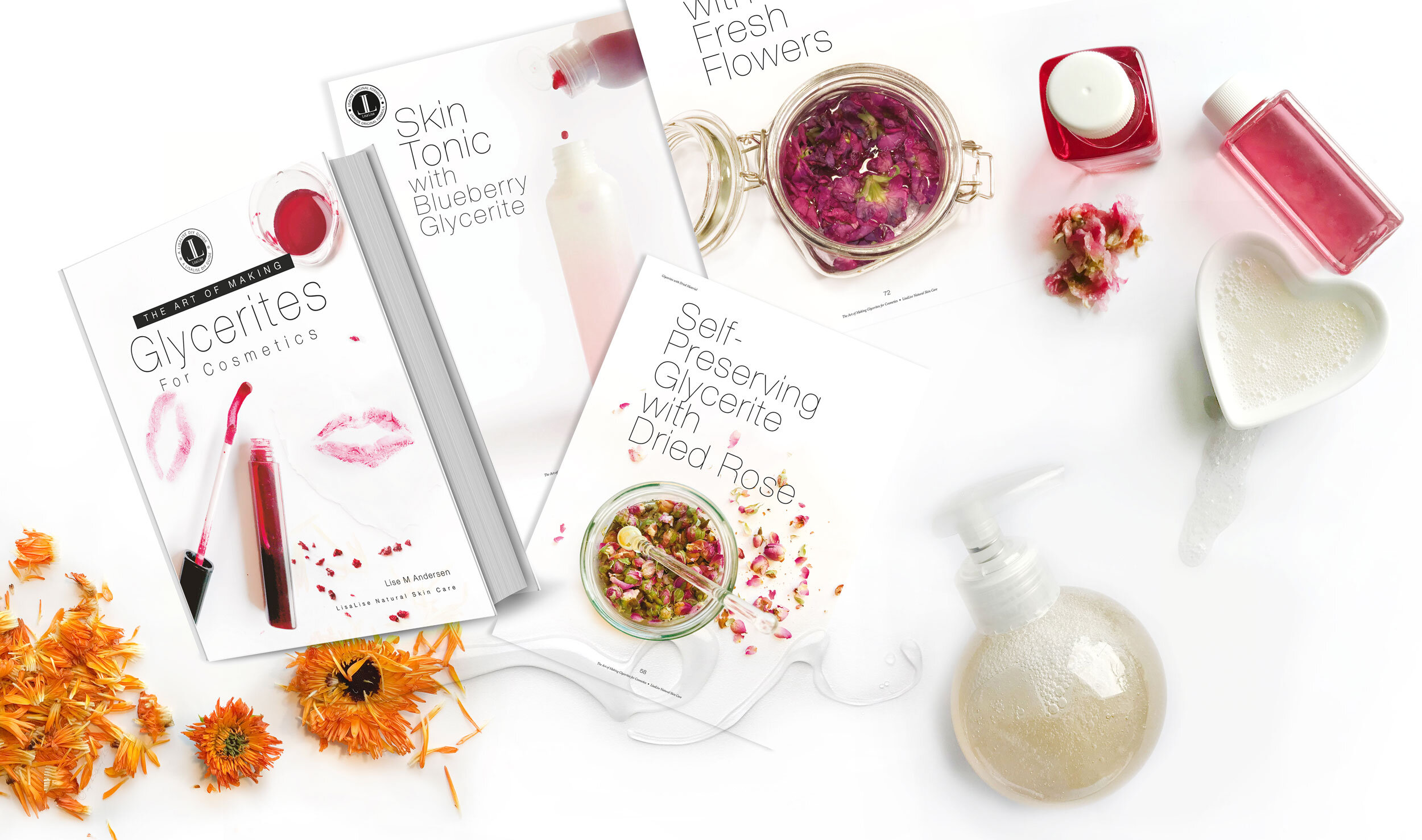The image features a collection of items centered around the theme of homemade cosmetics and glycerites. Prominently displayed are four white-covered books. The titles and images on the books are: "Glycerites for Cosmetics," featuring lip gloss and kiss mark images; "Skin Tonic with Blueberry Glycerite," showing a bottle pouring a pink liquid; "Self-Preserving Glycerite with Dried Rose," which has a jar with dried rose petals; and "With Fresh Flowers," depicting a mason jar with flowers submerged in liquid. To the bottom left, there are scattered orange dried flowers, while the top right corner hosts a smaller pile of dried flowers surrounded by colorful bottles filled with red liquid and capped in white. Nestled near these elements is a heart-shaped dish with a foamy mixture. Towards the bottom middle, a globe-shaped soap dispenser containing beige-yellow liquid adds to the specifics. The detailed imagery creates a cohesive and informative picture, emphasizing the books and surrounding items related to DIY glycerite cosmetics.